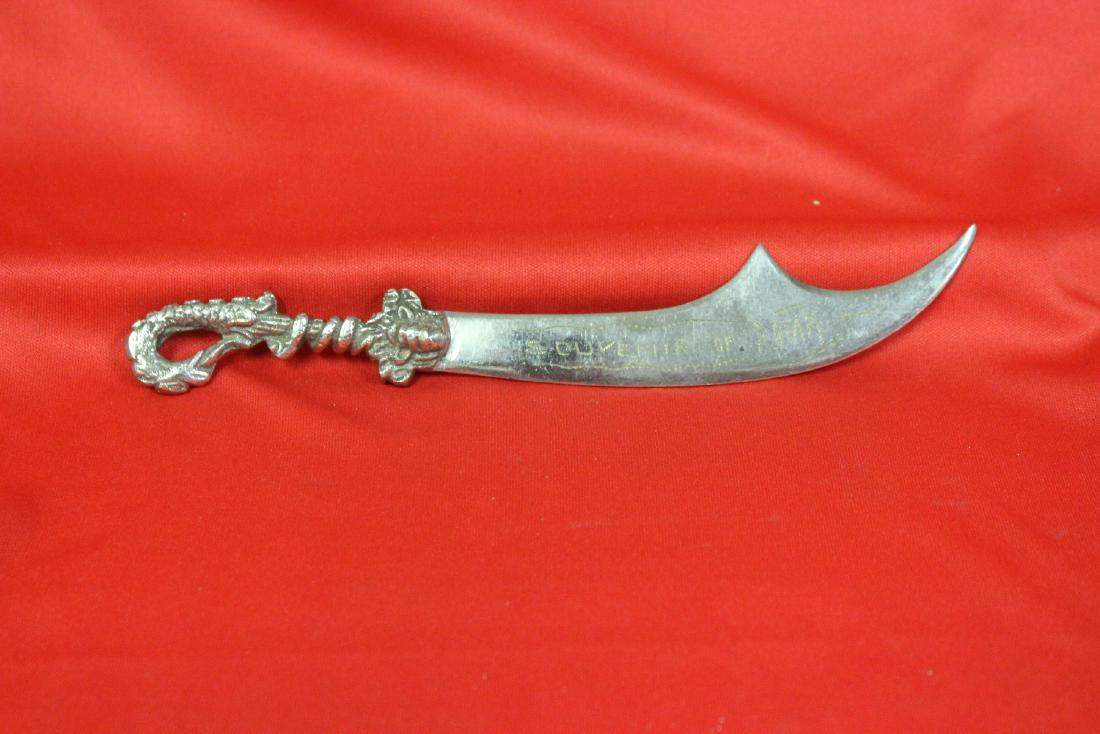The image showcases an antique, silver-colored weapon with a distinctly ornate design, lying atop a piece of vibrant, red satin fabric, possibly displayed in a museum setting. The weapon resembles a cross between a short sword and a knife, featuring a curved blade that forms two distinct points—one at the tip and another along its length. The handle is highly decorative, carved to resemble a fish or serpent, with a section seemingly being swallowed and its tail elegantly wrapped around the hilt, ending in an enclosed hook. Intricate engravings are visible on the blade, though the exact wording is unclear, it seems to hint at the term "souvenir," suggesting a memento. The red satin background beneath it appears slightly cushioned, adding to the display's opulent presentation.